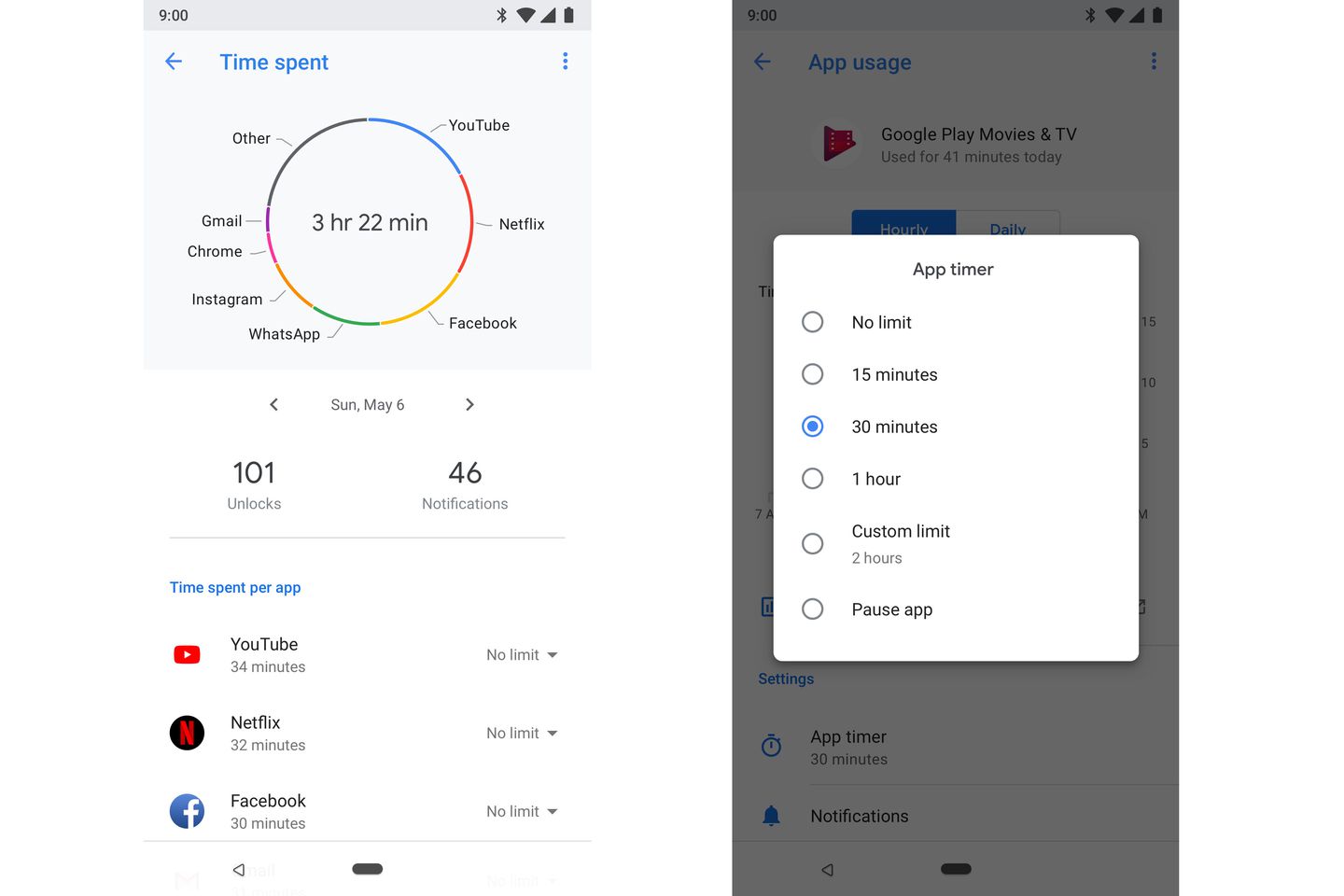In the image, there are two main sections divided into boxes. 

**Left Section:**
- **Upper Box:** 
  - Background Color: Light blue.
  - Top Banner: Darker blue with white text "9 o'clock."
  - Inner Light Blue Box: Contains the text "Time Spent" in blue print. There's a left arrow on the left side and three dots on the right side.
  
- **Middle Circle:**
  - A large, gradient-colored circle in the center, displaying multiple colors: blue, purple, orange, green, and red.
  - Icons inside the circle: Gmail, Chrome, Instagram, WhatsApp, Facebook, Netflix, and YouTube.
  - Center Text: "3 hours and 22 minutes" indicating total screen time.

- **White Box:**
  - Contains navigational arrows: left and right.
  - Text: "Sunday, May the 6th."
  - Stats: "101 unlocks, 46 notifications."
  - Below this, a gray line separates it from the next section.
  
- **Lower Section (large white box):**
  - Header in Blue: "Time Spent per App."
  - App Usage:
    - YouTube: 34 minutes, no limit (with a down arrow).
    - Netflix: 32 minutes, no limit.
    - Facebook: 30 minutes, no limit.
  - Below these app details, another gray line provides a visual separation.

**Right Section:**
- **Upper Box:**
  - Background color: Gray.
  - Top Text: "00".
  - Header in Blue: "App Usage" with a left arrow.
  - An icon resembling a small red flag with the text "Google Play, Movies and TV" indicating usage of "41 minutes today."
  - Little blue and white boxes: 
    - Blue Box: "Hourly."
    - White Box: "Daily."
    
- **Middle White Box:**
  - Header: "App Timer."
  - Options with Circles Next to Each:
    - No limit.
    - 15 minutes.
    - 30 minutes (highlighted in blue).
    - "1 hour," and a customizable limit of "2 hours."
  - Option: "Pause App."

- **Lower Gray Box (bottom):**
  - Headers:
    - "Settings."
    - "App Timer: 30 minutes."
    - "Notifications."
  - A left arrow provides a navigational option.

Overall, the image appears to be a detailed snapshot of a screen time management interface, showcasing various data visualizations and control options for app usage and time tracking.